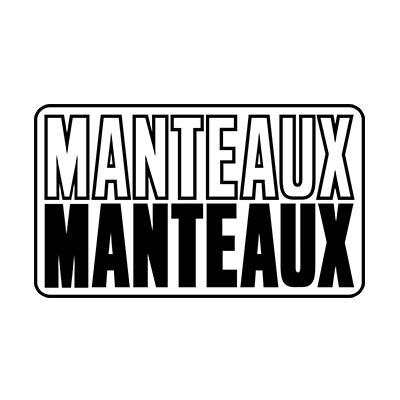The image depicts a rectangular box with rounded corners, placed against a fully white background. Inside the box, the word "M-A-N-T-E-A-U-X" appears twice, once in the top half and once in the bottom half. The top half displays the word in white letters with a thin black outline, while the bottom half features the same word in entirely black, filled-in letters. The white letters are contrasted against the transparent background within the box, making the black outline essential for their visibility. The black letters on the bottom half also stand out clearly against the transparent section. This repetitive typography suggests a mirrored but not completely symmetrical design, possibly serving as a logo or a graphic element.